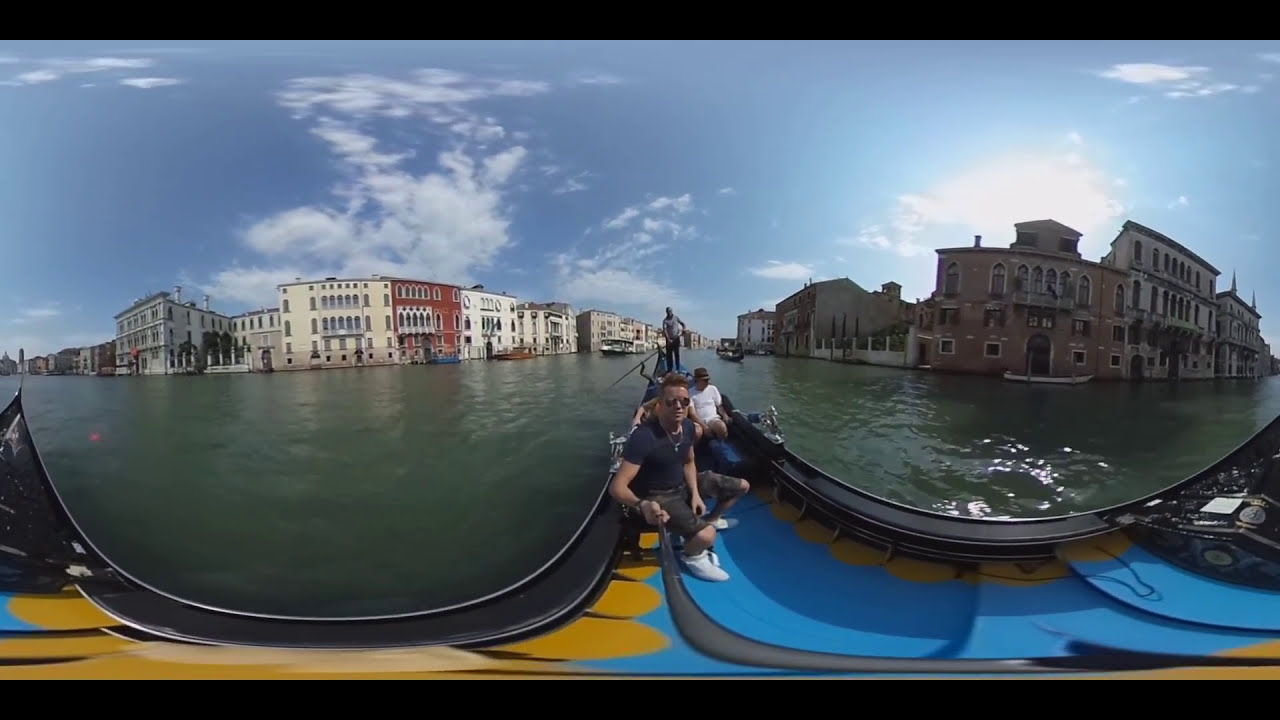This is a panoramic photograph capturing a vibrant scene along a canal in Venice, Italy. At the center of the image is a man seated in a gondola, holding a selfie stick to take a photograph. He is wearing a tight blue t-shirt, a necklace, black shorts, sneakers, and sunglasses, looking directly at the camera. The gondola’s interior features a bright blue and dark mustard color, creating a stark contrast with its black exterior. Due to the panoramic effect, the image of the gondola and the canal appears distorted, causing the canal to curve unnaturally around the scene. Behind the man, other passengers are seated, and at the bow, a gondolier stands, skillfully steering the gondola.

The canal is bordered by multi-story European buildings in a range of colors: white, red, dull yellow, and various earth tones. These buildings, typical of Venetian architecture, appear to be almost submerged in the greenish water of the canal. The background showcases a bright blue sky with clusters of white clouds and the faint glow of the sun peeking through. This outdoor scene beautifully encapsulates the essence of Venice by combining its unique waterways and historic architecture under a clear, serene sky.